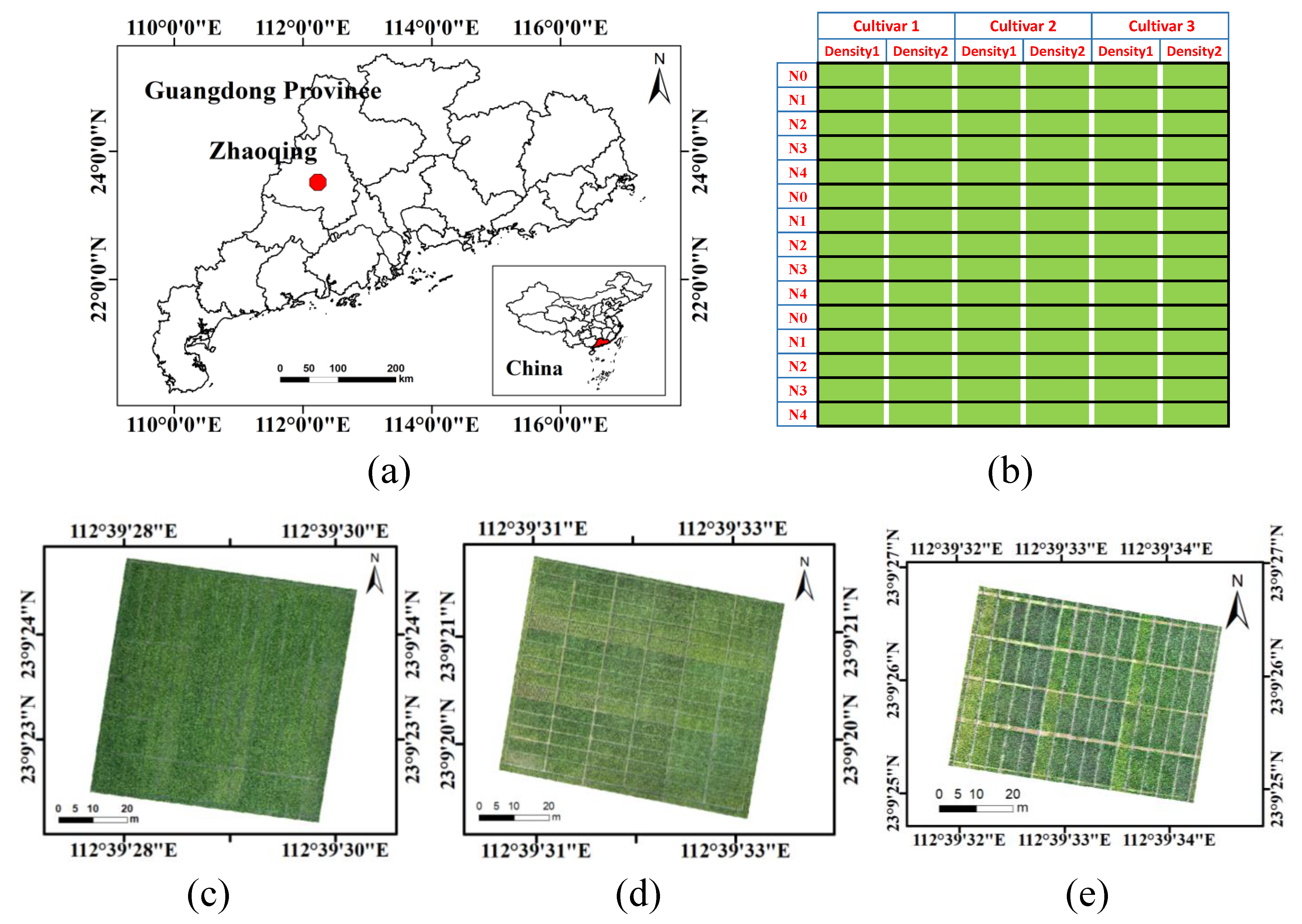The image is divided into five sections, with a map occupying the top-left corner. This map prominently features Guangdong Province, China, labeled in black and white. A large red circle marks the city of Zhaoqing. The map's borders display latitude and longitude coordinates, and a small inset in the bottom right corner shows the entire country of China, highlighting Guangdong Province in red.

Alongside the map, on the top right, is a detailed Excel spreadsheet. This spreadsheet is divided into three columns labeled "Cultivar 1," "Cultivar 2," and "Cultivar 3," each further divided into two sub-columns for "Density 1" and "Density 2." The rows are marked from 0 to 4, repeating for each cultivar section.

Below these top sections are three additional images, each displaying green square grids, suggesting farmland layouts. These grids are also annotated with latitude and longitude coordinates, similar to the map. The green grids within these squares are clearly defined and bright, making them easy to examine. Each of these sections, labeled A, B, and C, appears to represent different patches of land.